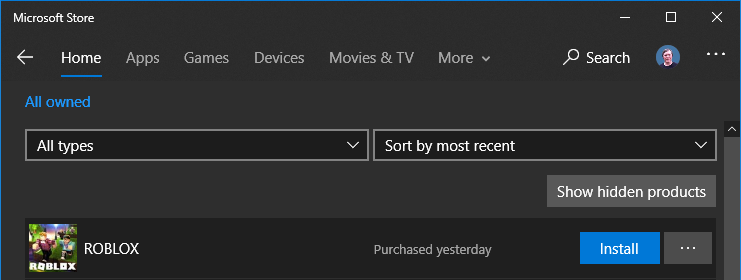The image features a black background with "Microsoft Store" written in white in the upper left corner. In the upper right corner, there are three icons: a minus sign, a square, and an 'X'. Immediately below, a navigation bar includes an arrow pointing left, the word "Home" underlined in blue, followed by tabs labeled "Apps," "Games," "Devices," "Movies & TV," and "More." To the far right, there's an image of a magnifying glass next to the word "Search" and a circular icon containing an image of a man with dark hair, wearing a t-shirt and smiling.

Further down, there's a blue tab labeled "All Owned." Below this, there are two rectangles: the first says "All Types," and the second says "Sort by Most Recent" with a downward arrow. Underneath these options, a light gray rectangle reads "Show Hidden Products." To the left of this section is an image titled "Roblox," showcasing blocky characters. To the right, a blue square features the word "Install."